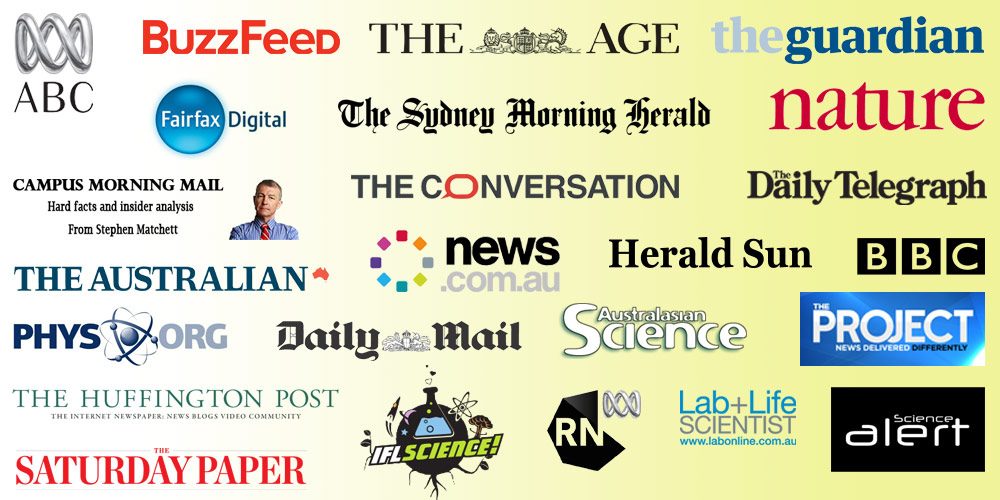The image showcases various media logos and a person. On the left, there is a "silver link" and the letters "B" and "C" in capital letters. Next to them, "BuzzFeed" is written in bold red letters, and below it, "The AGE" is in black. "The Guardian" appears in a combination of white, blue, and dark blue colors. "Fairfax Digital Fairfax" is depicted within a blue circle. "The Sydney Morning Herald" is written in black font. "Nature" is colored red. There is a headline reading, "Campus Morning Mail: Hard facts and insider analysis from Stephen Matchett," featuring an image of a man with brown hair. He is dressed in a blue collared shirt and a red-and-white striped tie. 

Additionally, "The Conversation" is mentioned with the letter "O" in red and the remaining letters in black. "The Daily Telegraph" is in black, while "The Australian" is written in blue. "News.com.au" is shown with multicolored squares. "Haraldson" appears in black font, followed by "BBC" in black. "FISE.org" is colored blue. "Daily Mail" is in black, and "Australia’s Science" is in white. Finally, "The Project: News Delivered Differently" is written with "News Delivered" in white and "Differently" in black.